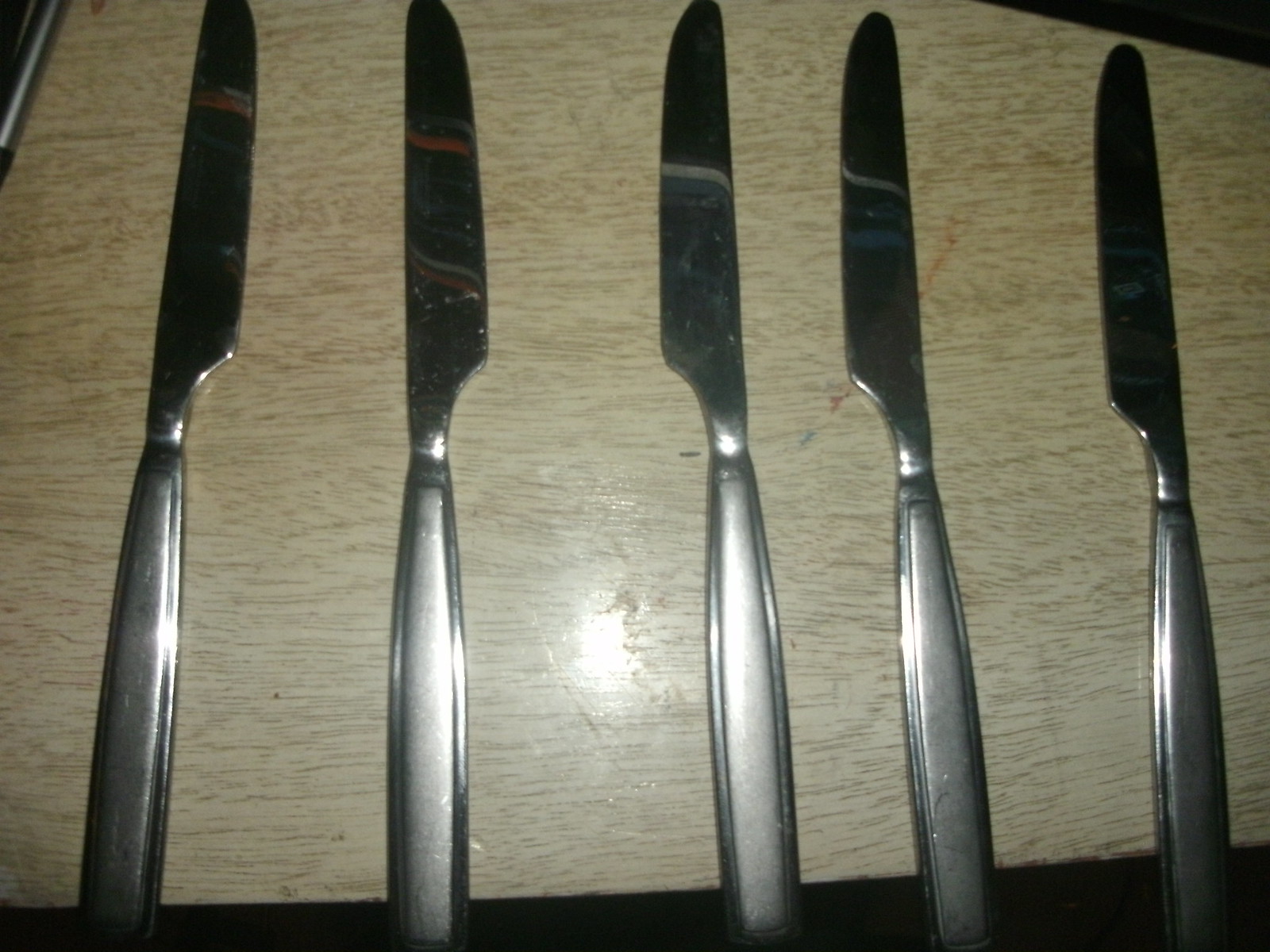The photograph depicts a row of five silver butter knives arranged on a slightly scuffed, gray, laminate table with dark brown wood grain patterns running horizontally. The first two knives on the left are oriented with their blades to the right, while the remaining three on the right are positioned with their blades to the left. The knives, which exhibit a generic and somewhat contemporary brutalist design, appear clean but slightly cloudy, possibly hinting at suboptimal polishing. The image is of amateur quality, with noticeable cropping issues that cut off both the tips and bottoms of the knives. There's a visible reflection of a light source between the second and third knives near the bottom of the frame, and faintly discernible colors like red, steel gray, and black are reflected on the knife surfaces. There are no additional markings, text, or date stamps within the image, and the table surface looks slightly dirty.